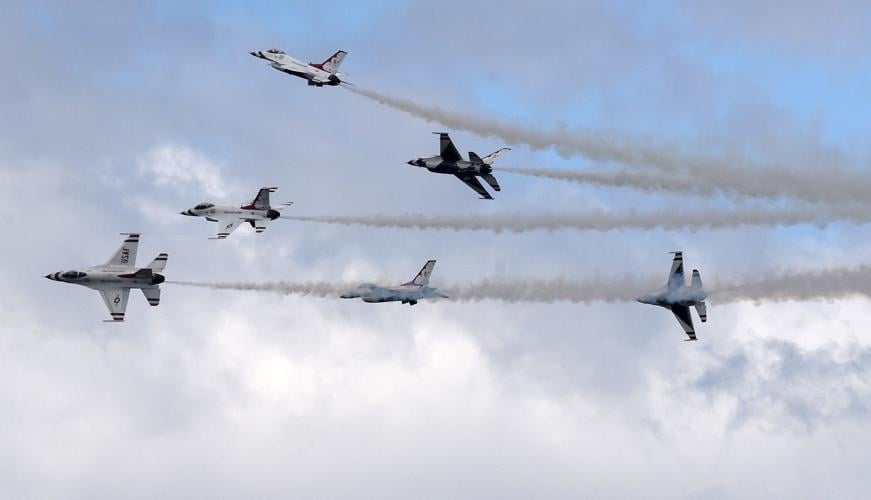The full-color photograph, taken outdoors during the daytime, features a horizontal rectangle without a border. The backdrop is a sky filled with clouds, with the upper portion appearing slightly clearer than the bottom, which is more clouded. The main focus is an air show where six white fighter jets are flying in formation. Each jet has visible contrails streaming behind it. Notably, one of the jets is inverted. The jets are arranged with three in a row and others distributed above and returning in the air. There are no people, buildings, or additional objects visible in the image.